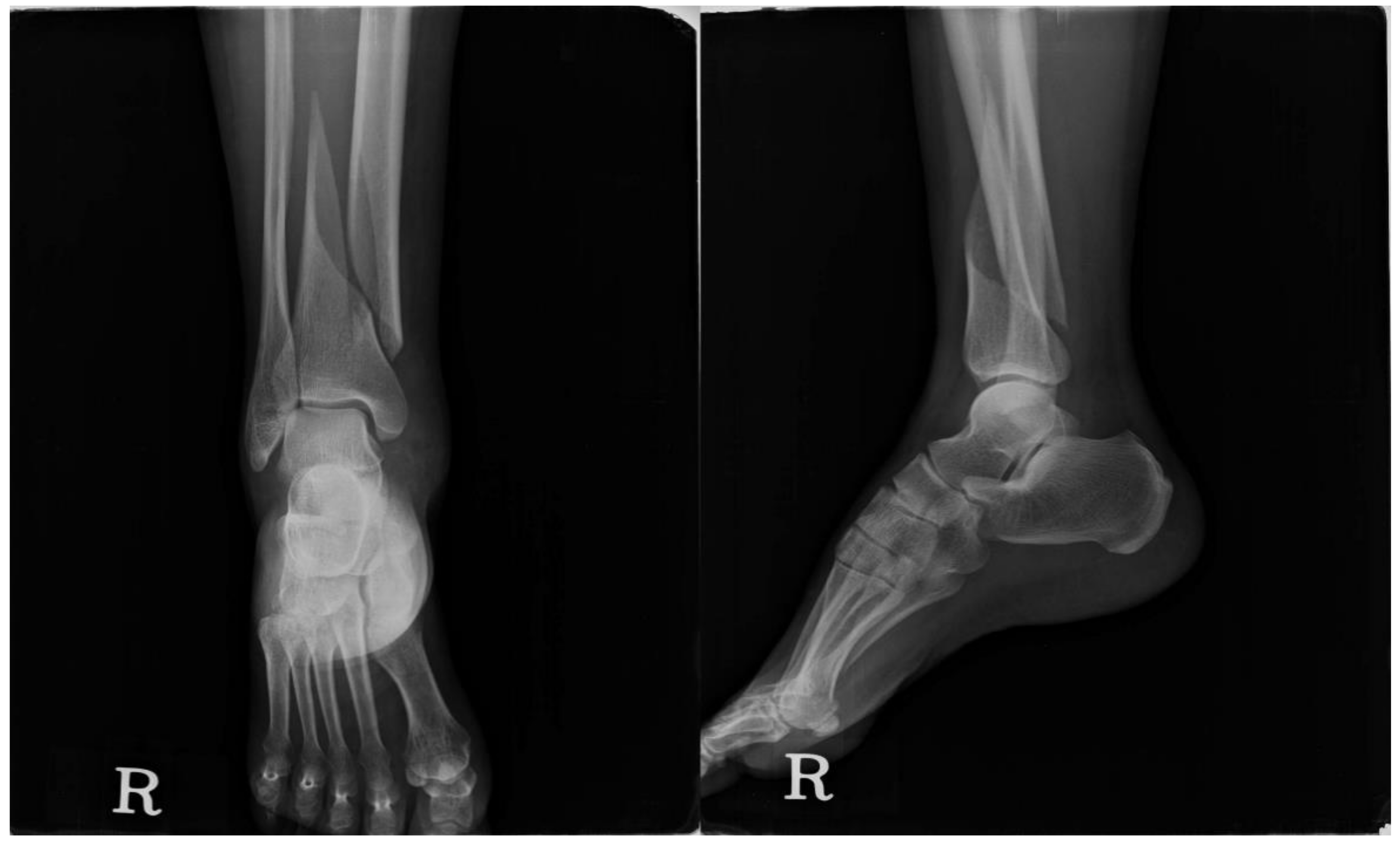This image displays two x-rays of the lower right leg and foot positioned side by side against a black background. Both x-rays are marked with a capital "R" in the lower left corner, indicating the right leg. The x-ray on the left provides a lateral view, capturing a side perspective of the foot, where the bones are predominantly white with varying shades of gray, and a faint gray patch visible in the top right corner. The x-ray on the right offers a top-down view, likely taken from above, showcasing the structure of the five toes and the joints, extending partway up the leg but not reaching the knee. Notably, there is a thin band of gray running along the top edge of this image. The bones appear pronounced against the dark background, creating a stark contrast that highlights the skeletal structure in detail.